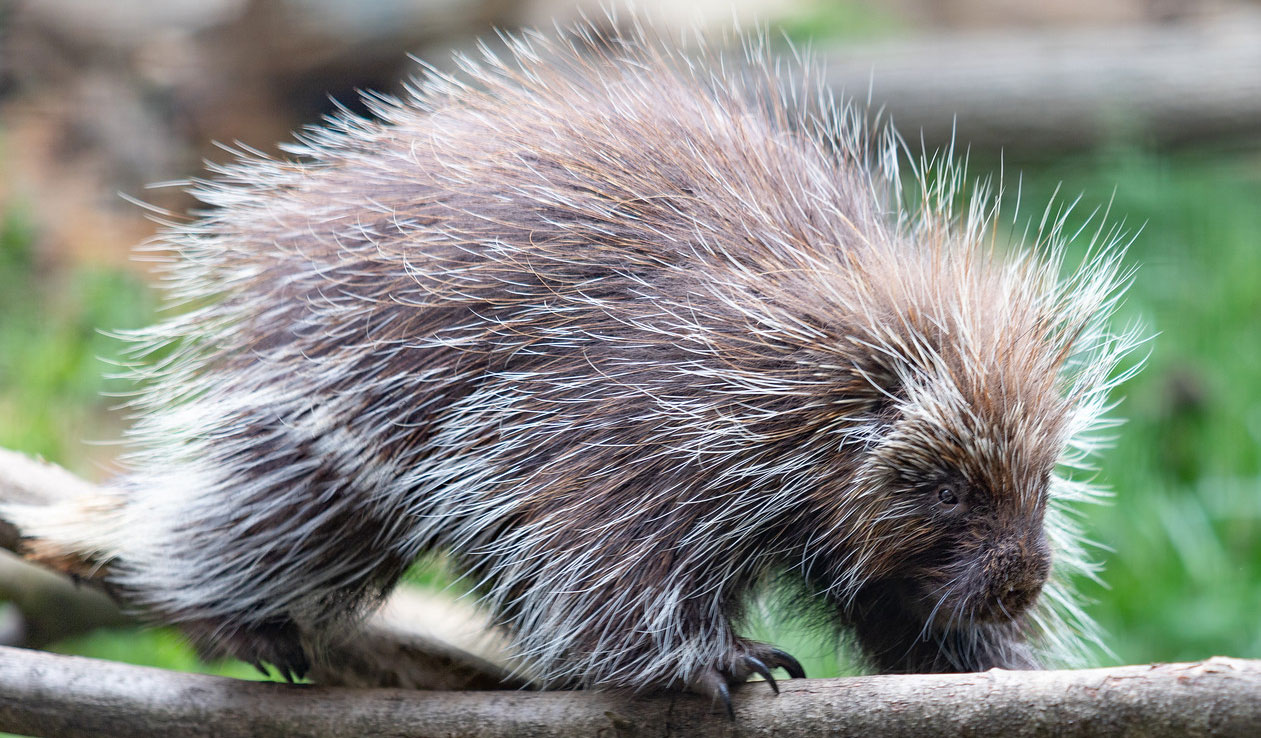This is a realistic, horizontal photograph taken outdoors during the day with ample natural light. The setting appears to be a forested or wooded area, characterized by out-of-focus green grasses and a possible fallen log in the background. The focal point of the image is a porcupine, positioned in the foreground on a light brown or grayish tree branch, which is about one to two inches in diameter and oriented horizontally across the scene. The porcupine, walking from left to right, has a predominantly brown coat with quills or hairs that transition to a grayish-white at the tips. Its small brown eyes are directed downward, and only its left front and left back legs are visible as they grip the branch with long claws. The details of the porcupine’s needles are clearly visible, standing upright, while the background remains a blurred mosaic of greens, oranges, and grays.